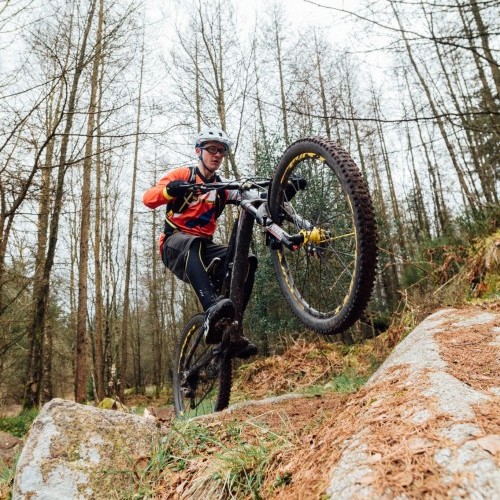The photograph captures an adventurous scene set in a forested wilderness during fall or winter, characterized by tall, barren trees with no leaves, revealing a white, cloudy daytime sky through their thin branches. The ground is covered in brown, dried grass, pine straw, and dead branches, indicating the season's transition. Central to the image is a white male cyclist, dressed in a white helmet, red long-sleeved shirt, and black shorts with black trainers, adorned with other protective gear including goggles. Mounted on a black bicycle, he is dynamically popping a wheelie to navigate over a small dirt hill amidst large stones. The predominant colors in the image include various shades of brown, green, yellow, red, black, and white, capturing the earthy and vibrant tones of the environment. Overall, the picture reflects the thrilling essence of an outdoor biking adventure.